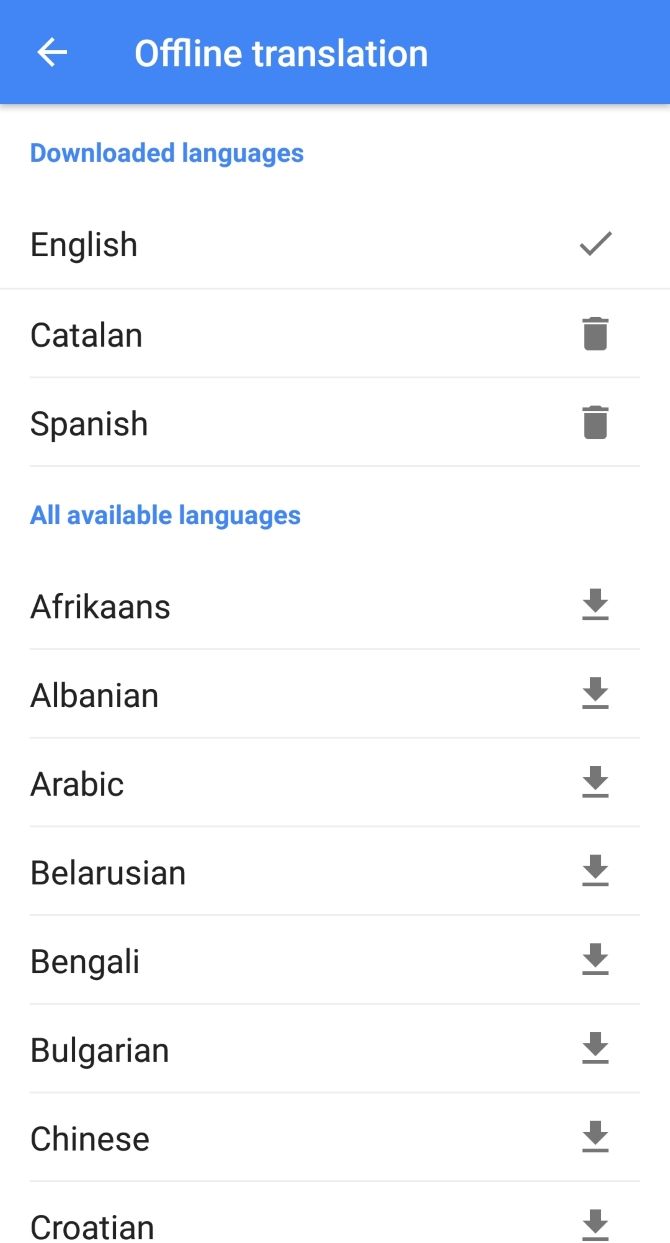A detailed screenshot of a language selection menu is displayed, specifically for offline translation purposes. The interface features a blue banner at the top, clearly marked "Offline Translation," with a left-facing arrow suggesting a back navigation option. Just below, the heading "Downloaded Languages" is prominently shown in blue text. Following this, the language 'English' is listed in bold black text, accompanied by a checkmark on the right, signifying its active or selected status. Underneath 'English,' there is a clear separation line followed by 'Catalan,' which features a trash icon on the right, indicating the option to delete this language. Another separation line appears below 'Catalan,' leading to 'Spanish,' which also includes a trash icon on the right and another separating line below.

Further down the interface, the text "All Available Languages" is displayed in blue, denoting the section for languages that can be downloaded. This section lists multiple languages: 'Afrikaans,' 'Albanian,' 'Arabic,' 'Belarusian,' 'Bengali,' 'Bulgarian,' 'Chinese,' and 'Croatian,' each followed by a separation line. To the right of each listed language in this section, there is a download icon with a downward-facing arrow, indicating the option to download these languages for offline use. The majority of the interface is set against a clean white background, providing a clear and uncluttered view of the options available. It is evident from the context that this list is part of an application or software, although it is not explicitly stated within the screenshot itself.